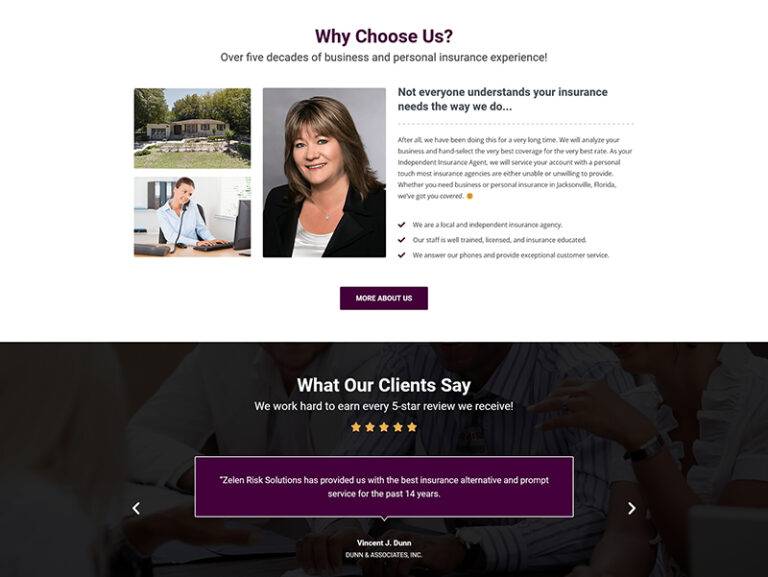### Caption for Business Screenshot Image

This detailed screenshot image for a business features multiple sections designed to convey the company's strengths and customer satisfaction. 

The top portion of the screenshot has a clean white background with bold purple print asking, "Why Choose Us?" Below this question, it states, "Over five decades of business and personal insurance experience." 

The middle section presents three images. The first two images are side by side:
1. A picturesque house set outdoors, surrounded by lush trees.
2. An office setting where a woman is seen multitasking, speaking on a cell phone while working on her computer.

Next to these, there's a professional headshot of a smiling woman dressed in a suit jacket, a white shirt, and a necklace. This image serves to personalize the service, reinforcing trust and professionalism.

Beneath the images, text states: "Not everyone understands your insurance needs the way we do." Though followed by a paragraph that appears somewhat blurred and hard to read, it likely contains additional supportive information about their services.

Further down, there are three bullet points with check marks, providing additional details on their offerings:
- "We are a local and independent insurance agency."
- "Our staff is well-trained, licensed, and insurance-educated."
- "We answer our phones and provide exceptional customer service."

A clickable banner labeled "More About Us" directs users to additional information. 

The bottom section of the screenshot switches to a black background and introduces client testimonials. It states, "What our clients say," followed by "We work hard to earn every five-star review we receive." 

Highlighted in a purple background is a testimonial that reads, "Zell and Risk Solutions has provided us with the best insurance alternative and prompt service for the past 14 years," accompanied by five stars, reiterating their commitment to excellent service and customer satisfaction.